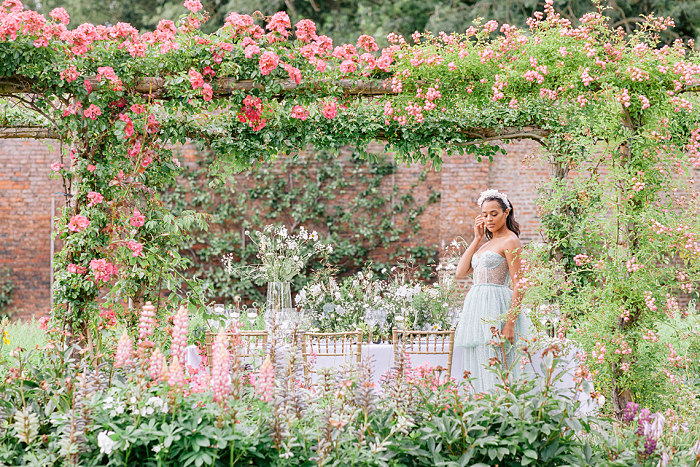In this outdoor photograph, a young woman, possibly a bride or bridesmaid, stands just off to the right of the center of the frame. She has long brown hair adorned with a white floral headband and is dressed in a strapless gown that appears to be a very light green, almost white in some lights. She poses gracefully with one hand lightly touching her cheek, her gaze directed downward. Surrounding her is a lush display of pink flowers and green leaves, creating a vibrant and abundant scene. These flowers form a rectangular arch around her, which is further accentuated by a background of climbing vines on a brick wall. In the foreground, a table covered with a white tablecloth and three light-colored chairs is partially visible but somewhat obscured by the floral abundance. The entire setting exudes an air of romantic elegance, with the floral elements dominating the scene.